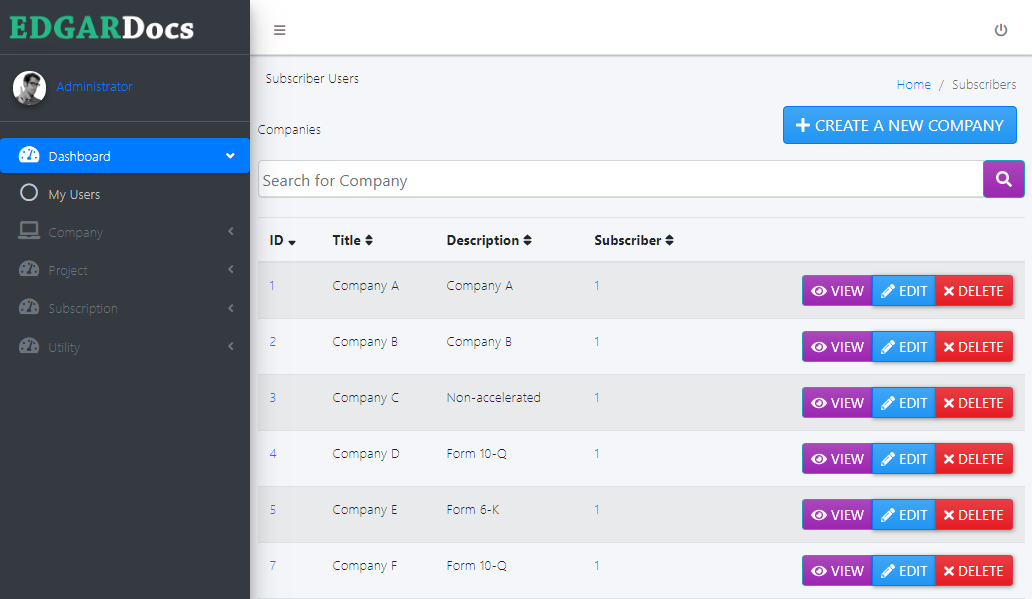The image is a detailed screenshot of a web page interface from a platform named "Edgar Docs," prominently displayed at the top in a blocky green font with the word "Docs" in white. The left sidebar features menu options in a vertical black column, starting with a black and white photo of a male administrator.

Below the photo are the menu options listed in white text: Dashboard (highlighted with a blue stripe), My Users, Company, Project, Subscription, and Utility. The main section of the page consists of a table displaying database records with alternating bands of dark green and light green, resembling a ledger.

Each row in the table is designated for different companies labeled from A to F, with columns for ID, Title, Description, and Subscribers. To the right of each row, there are actionable buttons: View (purple), Edit (blue), and Delete (red).

At the top of this data table, there are navigation options for subscribed users, home subscribers, and a search bar. Additionally, there's a prominent button to create a new company. The interface is structured to allow filtering and interaction with the database entries easily.